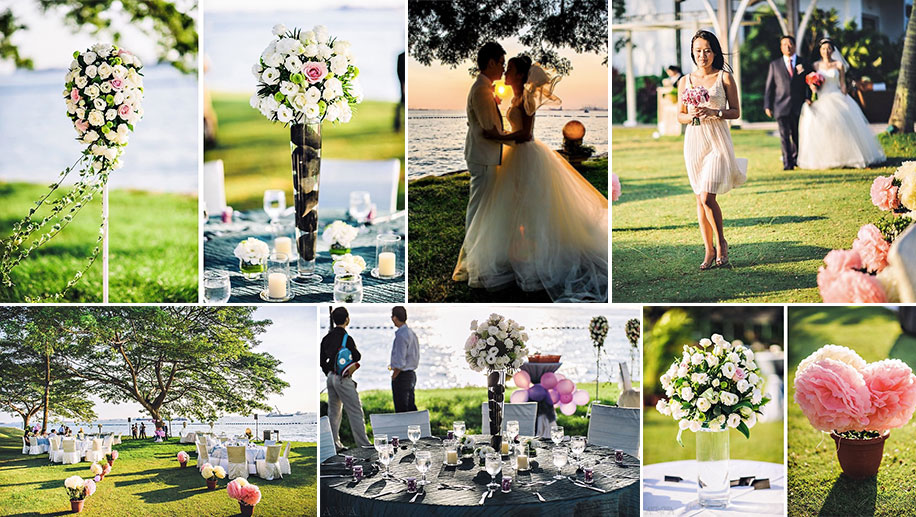This highly detailed photographic collage captures the essence of an outdoor wedding in daylight through eight horizontally arranged photographs. The top left panel features a bouquet of flowers fastened to a white pole set against a grassy field with a body of water in the background. Adjacent to it, a tall vase of flowers sits on a table surrounded by small tea light candles and single flowers in glasses. The third panel on the top row depicts a beautiful silhouette of the bride and groom, both dressed in white, sharing a moment under a tree with the setting sun and a serene lake in the background, enhanced by a red light to the bride's right. The fourth and final panel on this row captures a heartwarming scene with an Asian flower girl in a short dress, walking before the bride—who is in a long white dress and holding a bouquet of red flowers—being escorted by her father in a dark suit and red tie. A gazebo with arches and pink flowers can be seen behind them.

The bottom row, starting from the left, shows a picturesque setting of tables adorned with potted plants and flowers, situated on grass with people already seated, and a body of water framed by trees in the background. Next to this, another decorated table featuring the same tall vase of flowers from the top row, encircled by candles, single flowers in glasses, and showing a woman holding a blue pocketbook and a man in a white shirt and black pants gazing towards the water with balloons visible in the backdrop. The seventh panel on this row showcases a close-up view of a bouquet of white roses standing in a cylindrical vase on a table. Finally, the collage concludes with a potted plant displaying two large, vivid pink flowers. Overall, these images collectively convey the romantic and serene ambiance of the couple's memorable wedding day.